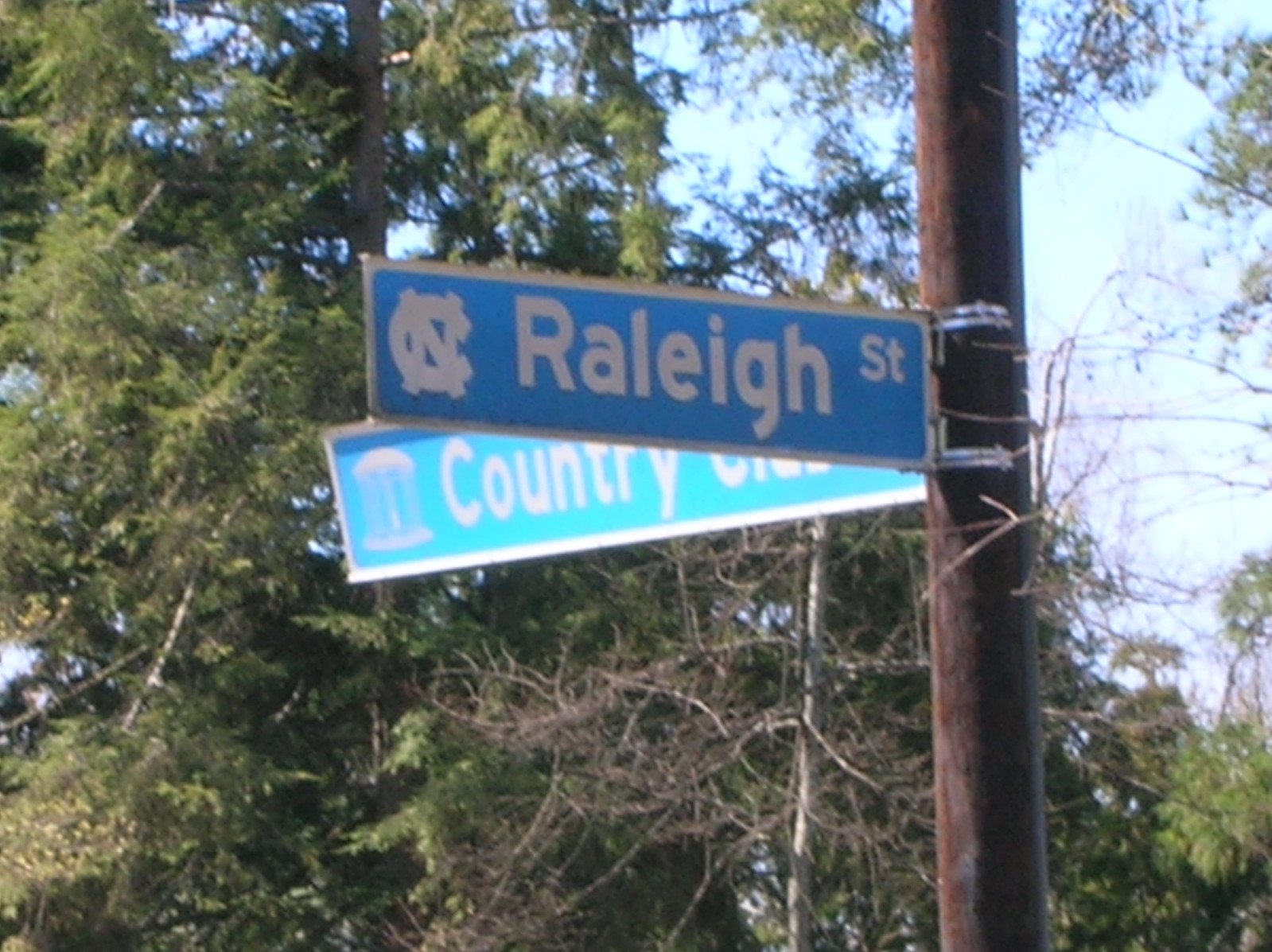The photograph is taken outdoors in what appears to be a rural or semi-wooded area, characterized by tall trees that extend from the middle left to the bottom of the image, creating a mostly green and leafy background. A blue sky peeks out in the right-hand corner of the image. Dominating the foreground, a wooden pole runs vertically from the bottom to the top of the picture. Attached to this pole are two blue street signs: the top sign, facing left, reads "Raleigh ST" with a distinctive 'C' and 'N' graphic; the lower sign, partially obscured by the top one, seems to read "Country," but the rest of the word is cut off. The blue signs with white borders are positioned perpendicularly to each other, making a right-angled intersection.